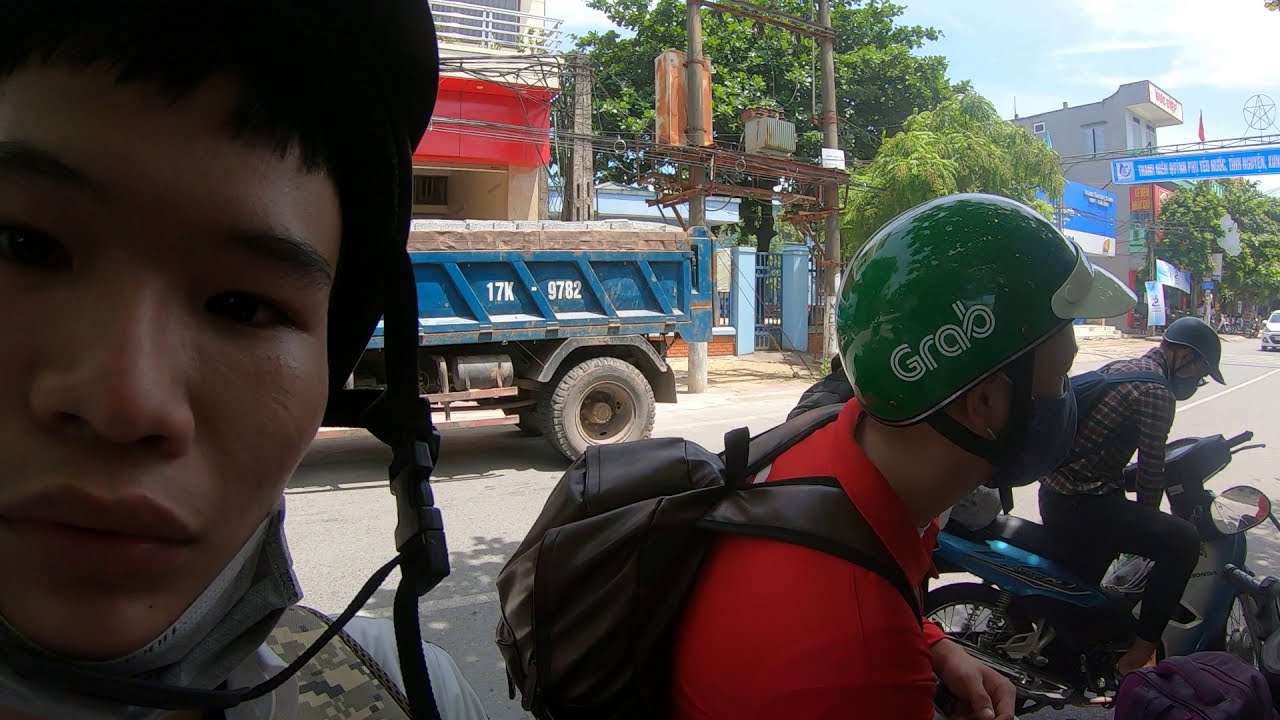The image depicts a vibrant street scene in an Asian city, featuring several individuals seated on motorcycles or scooters near various buildings. Prominently in the foreground to the left is a man of Asian descent, who appears very close to the camera and displays a blank expression. He has short black hair and is wearing a helmet. To his right, there are at least two more people on bikes. One person, positioned centrally, is adorned with a black backpack, a green helmet branded 'Grab', a red shirt, and a face mask. Another person further right, slightly distanced, is seen in a plaid shirt, black jeans, dark green helmet, face mask, and glasses, sitting on a motorcycle with bright blue metallic parts.

In the background, a dump truck with a blue bed and identifiable code 17K 9782 is visible, along with a building with a red awning. Additionally, a street sign with Latin letters in an unfamiliar language is seen, indicating the location's Asian context. The scene is also dotted with power transformers on poles and a few trees, all under a bright blue sky with scattered white clouds.